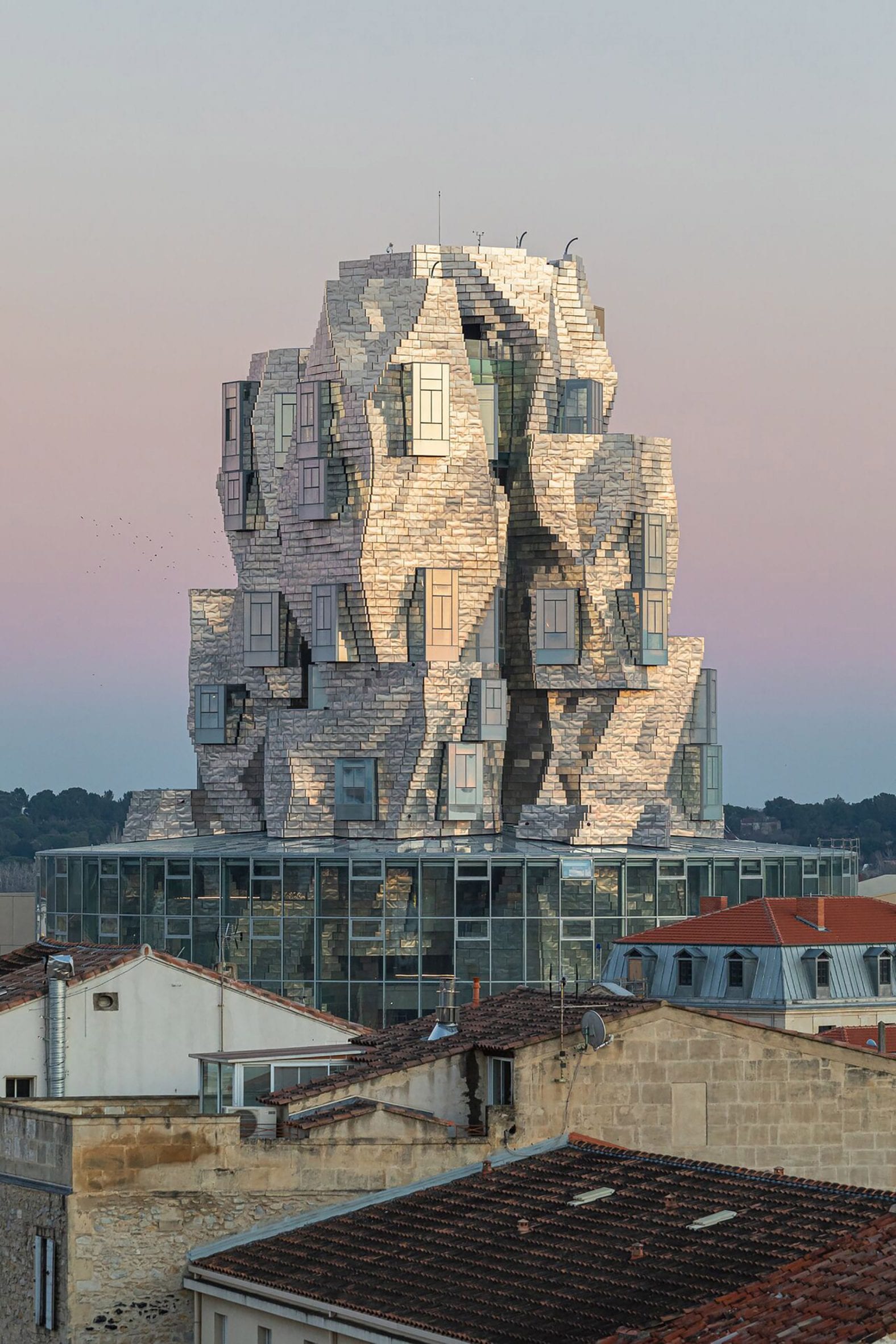This vertical portrait image, captured outdoors during the day, showcases a striking, multi-storied stone building that dominates the center. The sky features a beautiful gradient of light purple, blue, pink, and grey tones. The building itself is constructed from a combination of white and grey stones, reminiscent of a retaining wall, giving it a robust yet elegant appearance. The windows are uniquely staggered, positioned at various levels and angles, defying the conventional alignment of floors. 

The lower portion of the building is characterized by a flat-roofed section, clad in silver or grey, with multiple vertical rectangular windows. Beneath the main structure, the rooftops of older buildings extend from left to right. Notably, an older stone building with a light brown color and a matching brown roof is visible towards the middle, alongside a roof with distinctive red tiles and adjacent worn brown tiles in the lower right corner. This tall, futuristically-designed building, possibly computer-generated, stands out against the eclectic mix of older rooftops, culminating in a vivid and engaging urban scene.